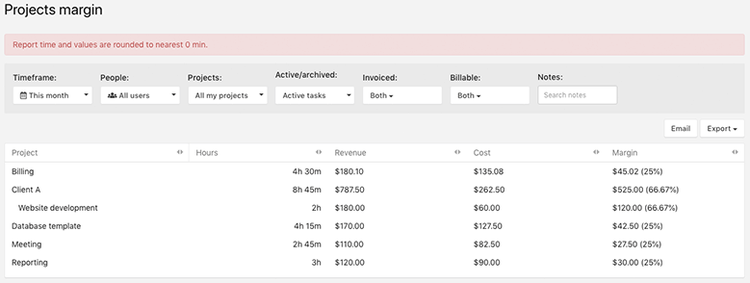**Detailed Descriptive Caption:**

This image is a detailed screenshot captured from a spreadsheet or investment/billing software, specifically focusing on project margin analytics. The title of this section is prominently labeled "Projects Margin." The interface includes multiple drop-down menus allowing for filtering based on timeframe, people, projects, archiving status, invoiced items, billable status, and notes.

The spreadsheet section is organized with several columns: Project, Hours, Revenue, Cost, and Margin. Each column meticulously lists relevant data. The topmost entry under the Project column is "Billing," which details a work duration of 4 hours and 30 minutes, revenue amounting to $180.10, a cost of $135.08, and a resultant margin of $45.02, translating to 25%.

Following this, the spreadsheet continues with other projects such as "Client A," "Website Development," "Database," "Tablet," "Meeting," and "Reporting." Each of these projects displays unique figures for hours worked, revenue generated, costs incurred, and the corresponding profit margins.

The values are rounded to the nearest minute for precise reporting, supporting clear and concise interpretation of the financial data related to each project. This structured layout enables users to efficiently analyze the financial performance and margins of various ongoing and past projects.